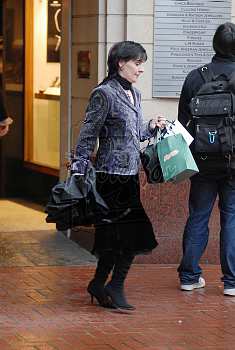The photograph captures a candid scene of a woman and a man standing on a reddish-brown brick or tile pedestrian pathway, possibly near a shopping area. The focal point is a full-length profile of the woman, who is dressed in a light gray denim-style jacket that is closed, a black skirt extending below her knees, and high stiletto-heeled boots reaching up to her knees. She has short black hair, pulled back into a ponytail, and light skin. Around her neck is a black scarf. She carries multiple small green paper bags with handles in one hand and a folded black umbrella in the other.

To her right, a man dressed in a black jacket, blue denim jeans, and white sneakers stands facing away from the camera, his backpack visible, gazing at an unclear sign. The background includes an open doorway to a building, contributing to the casual, candid nature of the photograph. The color palette of the image includes black, white, peach, pink, gray, brown, red, yellow, and gold, enhancing the detailed and spontaneous atmosphere.